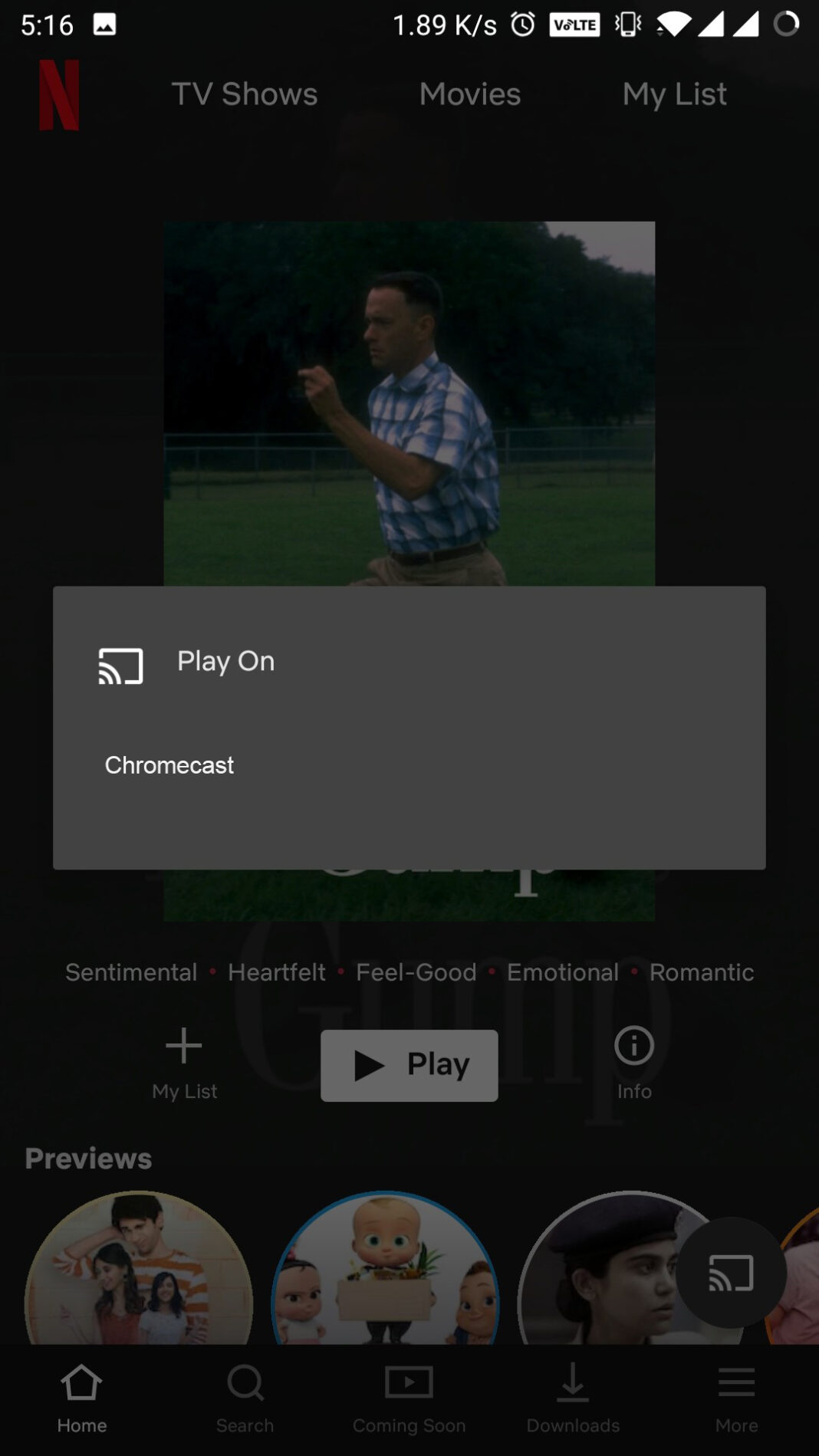The image showcases the Netflix mobile app interface. In the upper left corner, the iconic red Netflix logo is prominently displayed. To the right of the logo, there are three tabs in white text: "TV Shows," "Movies," and "My List." Below these tabs, a still from the movie "Forrest Gump" is featured, capturing the iconic scene where Forrest is running. This image is accompanied by descriptive tags such as "Sentimental," "Heartfelt," "Feel-Good," "Emotional," and "Romantic."

Directly beneath the movie scene, there's a row of options with a plus symbol on the left to add the movie to "My List," a central play button in white and black, and an info button on the right. Further down, there's a "Previews" section with icons representing various movies.

At the very bottom of the screen, there are navigation tabs labeled "Home," "Search," "Coming Soon," "Downloads," and "More." Dominating the center of the image is a gray pop-up box that reads "Play On," offering the option to stream the movie to Google Chromecast.